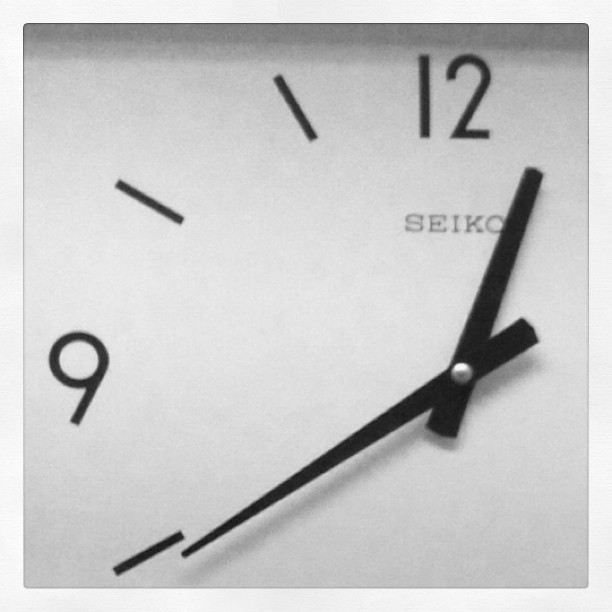This black-and-white square photograph is an extreme close-up of either a clock or a watch face. The image features a very thin gray frame on the outside, followed by an inner razor-thin black frame. The picture primarily shows the segment of the timepiece from the 8 to the 12. The face is plain white, and the hands are simple: the hour hand is a blunt, thin rectangle, while the minute hand is a long strip ending in a point, indicating the time as 20 minutes to 1. The brand "Seiko" is written in black ink under the number 12. The numerals 9 and 12 are visible, along with three black dashes on the face. A shadow, darker than the white face, shades the upper part of the image. The extremely close perspective makes it challenging to determine whether the timepiece is a watch or a wall clock.